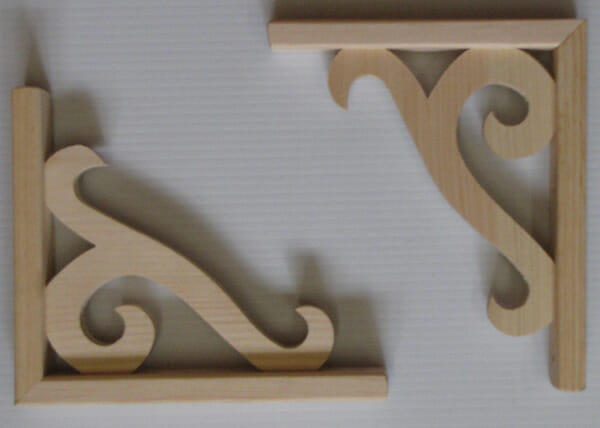The image is a square photograph featuring two intricately designed wooden objects positioned diagonally: one in the lower left corner and the other in the upper right corner. These objects appear to be ornate wooden brackets, possibly used as bookends or decorative shelves. They are made from light-colored, unstained wood and each piece is crafted into an L-shape with a curvilinear pattern reminiscent of a fancy 'S' or 'Y', with elegant swirls connecting the straight edges. The background is a subtle beige with gentle horizontal lines, adding a soft, muted tone to the overall image. The wood grain is visible, with the piece in the upper right showing vertical grains and the one in the lower left displaying horizontal grains. Shadows cast by the objects suggest they are resting flat against the surface. The photograph is taken indoors, likely on a table, capturing a detailed and closely-framed view of these decorative wooden pieces.